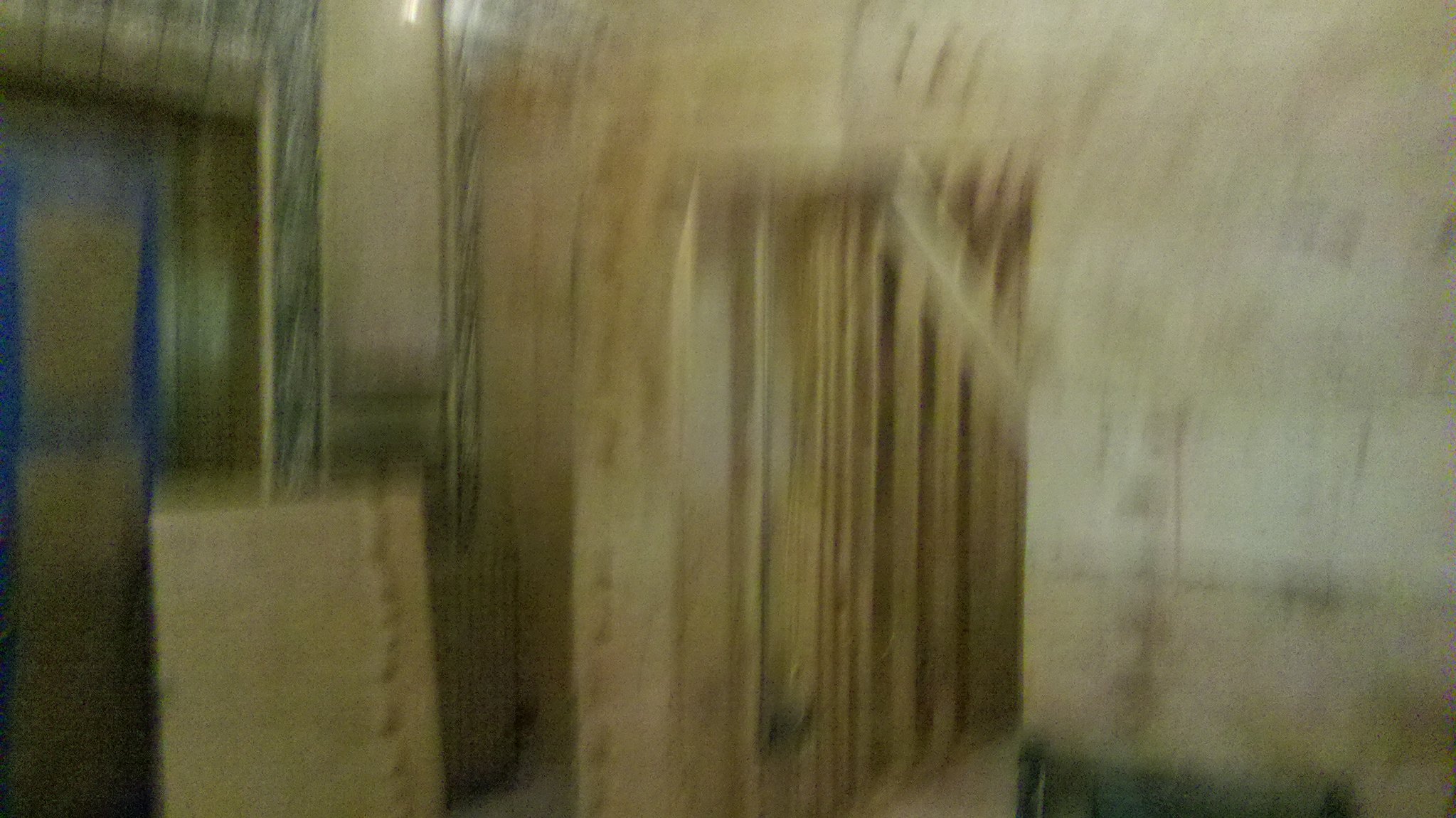This horizontally rectangular image, despite its extreme blurriness, offers a glimpse into the interior of a structure currently under construction. On the right side and top of the frame stands a large cinder block wall that prominently features a doorway opening. Beyond this doorway, one can discern the placement of dimensional lumber studs, indicating preparations for subsequent drywall installation. On the left side, a potential second doorway can be observed, distinguished by a grayish marble border that adds an element of sophistication amidst the raw, unfinished construction environment.